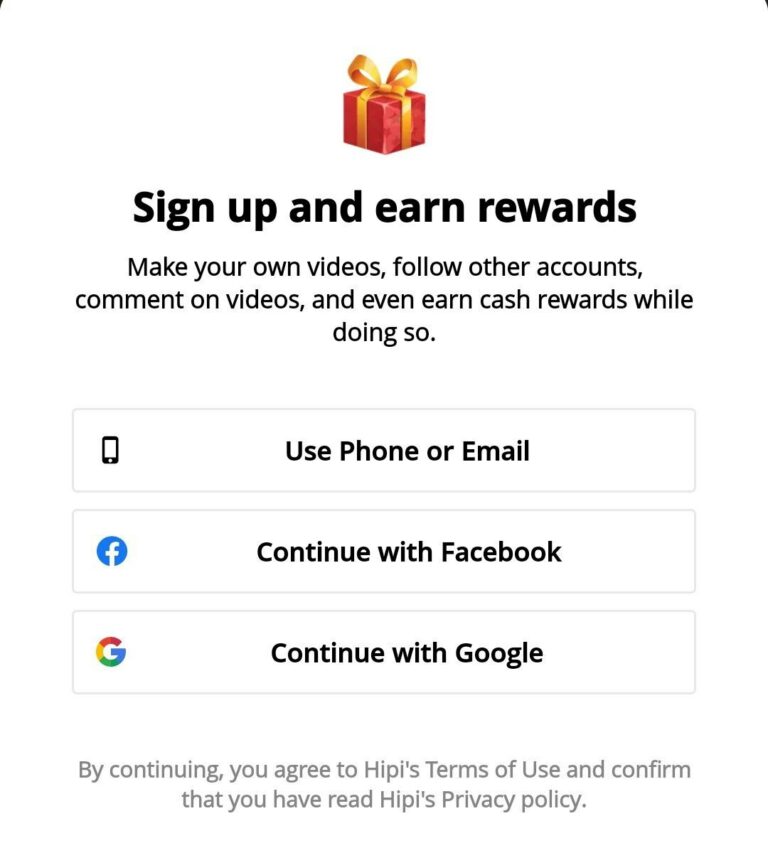On a pristine white background, a visually striking, gift-wrapped red present adorned with a lustrous golden-orange bow is prominently displayed at the top center. Beneath this appealing image, the text "Sign Up and Earn Rewards" is boldly presented in large black letters. Further below, in smaller, non-bolded text, the caption elaborates: "Make your own videos, follow other accounts, comment on videos, and even earn cash rewards for doing so."

Following this informative section, a white rectangular input field with a subtle gray border appears. Within this box, the prompt "Use Phone or Email" is clearly indicated next to a miniature cell phone icon positioned on the left. Below this entry field, there is another identical white box, featuring a Facebook icon on the left and the option to "Continue with Facebook." Another similar box follows, this time displaying the iconic Google 'G' logo on the left and the text "Continue with Google."

At the bottom of these options, a disclaimer in gray text reads: "By continuing, you agree to Hippie's Terms of Use and confirm that you have read Hippie's Privacy Policy." The remainder of the space is a clean, unoccupied expanse of white, contributing to a clutter-free and visually appealing layout.